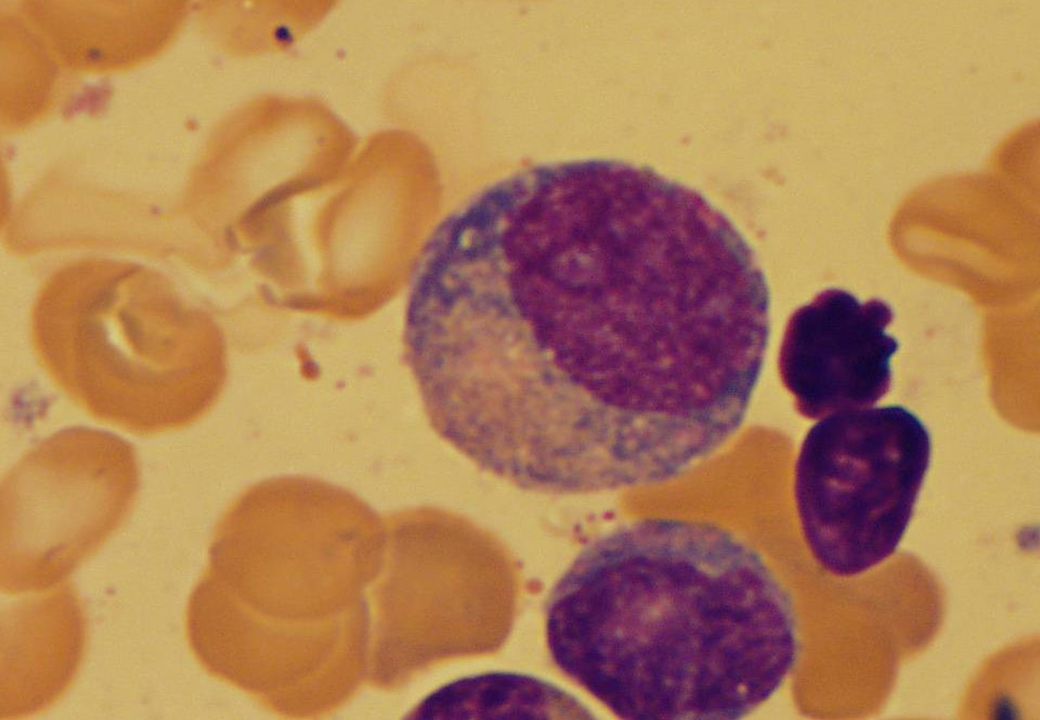The image presents a close-up microscopic view of various cells on a yellow-tan background. The cells are stained in different colors; most notably, there are several prominent round to oblong purple cells, each containing a darker purple inner circle. Surrounding these purple cells are clusters of smaller orange cells, interspersed with tiny purple and orange dots. The scene resembles an abstract pattern, resembling a late 1960s ink show, with the purple, brown, and yellow hues blending in a visually dynamic composition.